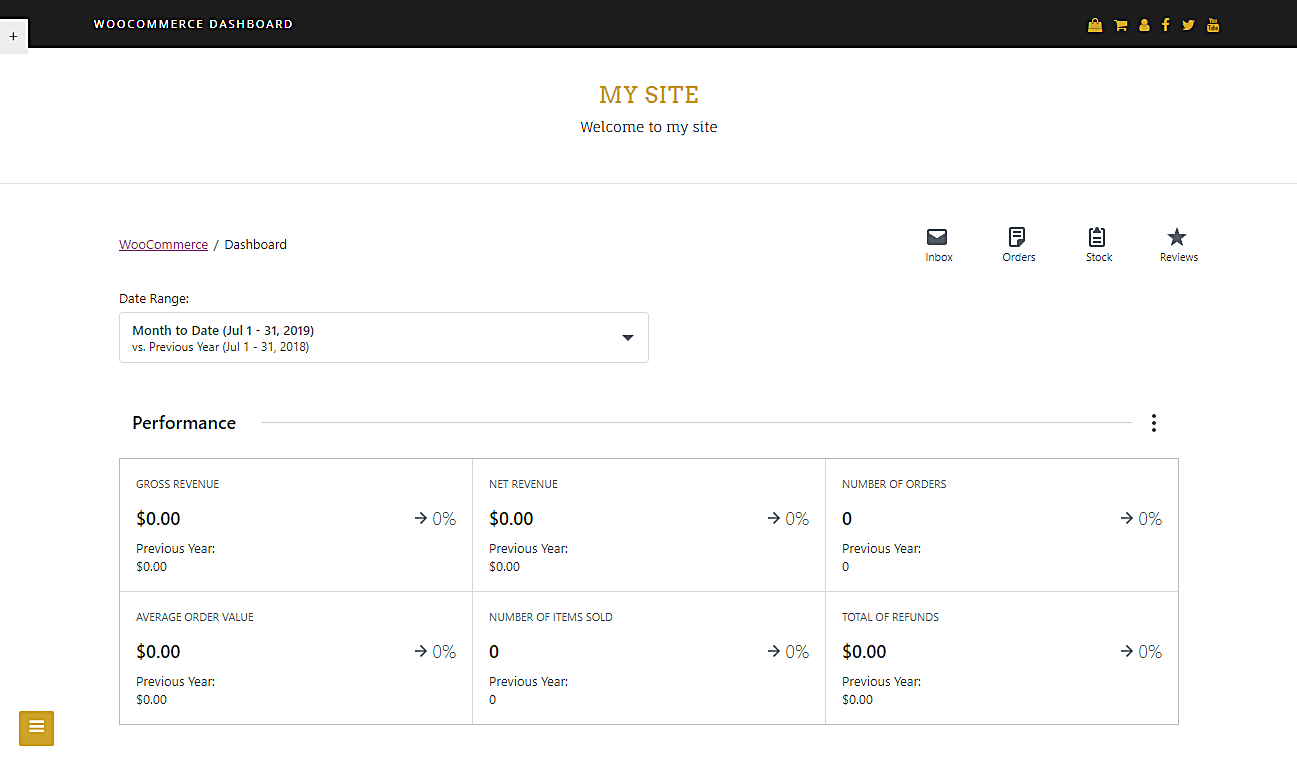### Detailed Screenshot Description of an Online Web Design Page for an Established WooCommerce Site

The screenshot is of an online web design page for a WooCommerce site, showcasing the WooCommerce Dashboard. The top section of the screenshot features a black data bar. On the upper right-hand corner of this black bar, "WooCommerce Dashboard" is displayed in white text. On the opposite side of this bar, there are six gold-colored icons.

Directly below this black bar is the main section of the screen. The words "My Site" are prominently displayed in gold text, followed by "Welcome to My Site" in smaller black text. Below this welcome message, there is a purple-highlighted link that reads "/dashboard," indicating the current active page under WooCommerce.

On the far right side of this dashboard section, there are four selectable icons labeled: "Inbox," "Orders," "Stock," and "Reviews."

Beneath this dashboard summary, there is a small rectangular window titled "Date Range," which allows users to specify a time frame for their data. Below the date range window, options such as "Month to Date" and "Versus Previous Year, Same Date Range" are available for selection.

The main content area of the screen is titled "Performance." This area contains six distinct sections, each with corresponding metrics:
1. **Gross Revenue**
2. **Net Revenue**
3. **Number of Orders**
4. **Average Order Value**
5. **Number of Items Sold**
6. **Total Refunds**

Currently, all the values in these fields are set to zero, indicating that no activity has been recorded yet. 

This detailed arrangement provides a comprehensive overview of the WooCommerce dashboard, facilitating effective site management and data analysis.